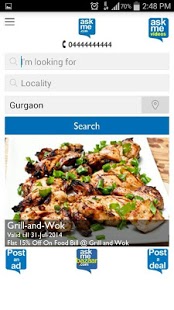The image shows a smartphone screenshot taken at 2:48 PM with a battery level of 70%. The top left corner of the screen features a hamburger menu icon. Prominently displayed in the center is an image of a grilled chicken dish. Below the image, there's a search bar with a magnifying glass icon next to the text "Gurgaon," indicating a search for local deals. 

The content includes an advertisement for "Grill and Wok," offering a flat 15% discount on the food bill, valid until January 31, 2014. At the bottom of the screen, there are various interaction options labeled "Post-Ad," "Ask Me," and "Post Deal." The entire interface is set against a clean, white background.